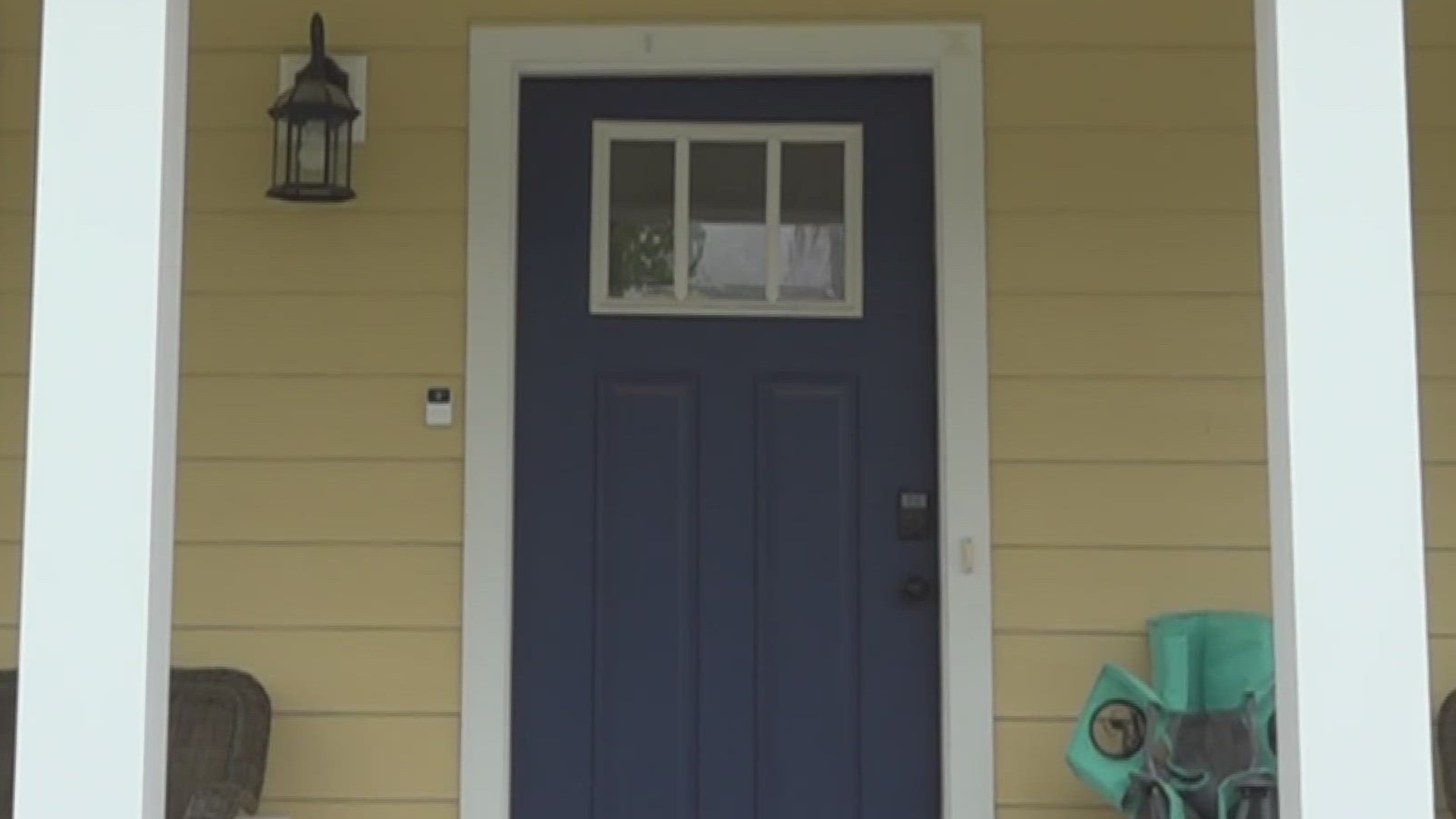This detailed photograph captures the charming front porch of a house. Central to the image is a dark blue front door adorned with a white-framed window consisting of three panes. A black knob with a keypad entry lock is visible on the right side of the door. The door is encased in a white border, and the house itself features yellowish-brown wooden siding. Flanking the entrance are two white vertical columns. To the left of the door, a black lantern-style porch light with a white bulb hangs, casting a downward glow. Additionally, there is a doorbell situated on the white frame of the door to the right. The porch is decorated with two seats—a brown chair to the left, and a vibrant lime-colored chair to the right. Overall, the image reflects a well-maintained and inviting entryway bathed in natural daylight.